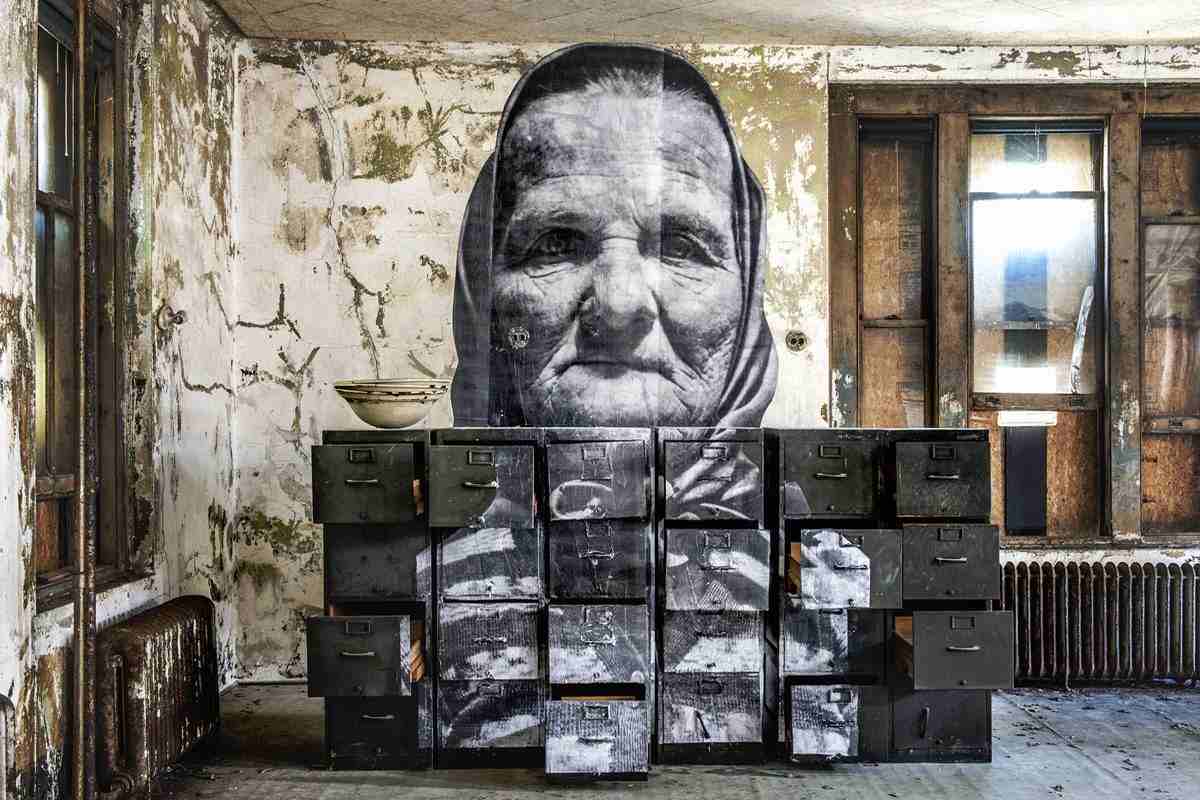The image showcases an art piece set inside a dilapidated building with green, cracked, and peeling walls. The setting includes multiple deteriorating elements, most notably two dingy, rusted radiators located beneath two old wooden windows—one on the left and the other on the right. The worn wooden floors have a grayish-green texture. Central to the scene is a row of metal file cabinets, each with four drawers, painted dark green. Some drawers are ajar, while others remain closed. An intriguing element of the artwork is a realistic black-and-white image of an elderly woman wearing a headscarf, extending from the wall behind and seamlessly continuing onto the fronts of these cabinets. The woman's face, framed by the headscarf, gazes outward with a haunting presence. Adjacent to the right of the cabinets, beneath another old window, rests a large bowl in shades of tan, white, and brown, further adding to the layered textures of decay and artistry evident throughout the room.